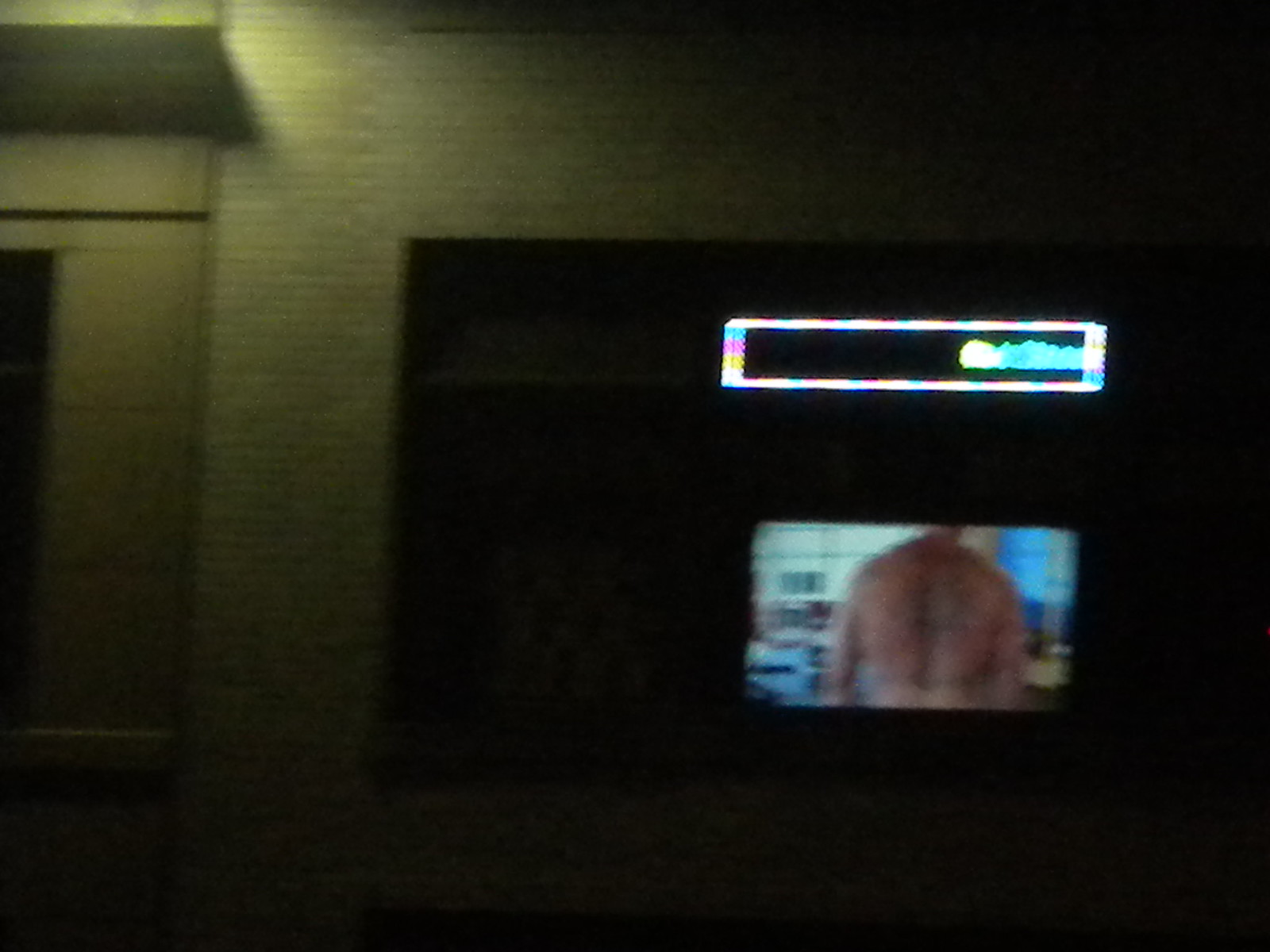An unfocused and dimly lit photograph captures a section of a wall adorned with green fabric-like wallpaper. Towards the center-right of the image, there is a flat panel, possibly a TV, displaying an unclear image. The left side of the photograph hints at either another TV or a window, though it is too dark to distinguish. The right side of the frame fades into complete darkness. On the TV screen, which occupies a dark area of the wall, a small illuminated portion reveals what seems to be a man's back, possibly showcasing a tattoo or another indistinct element. The overall scene is shrouded in ambiguity due to poor lighting and lack of focus.